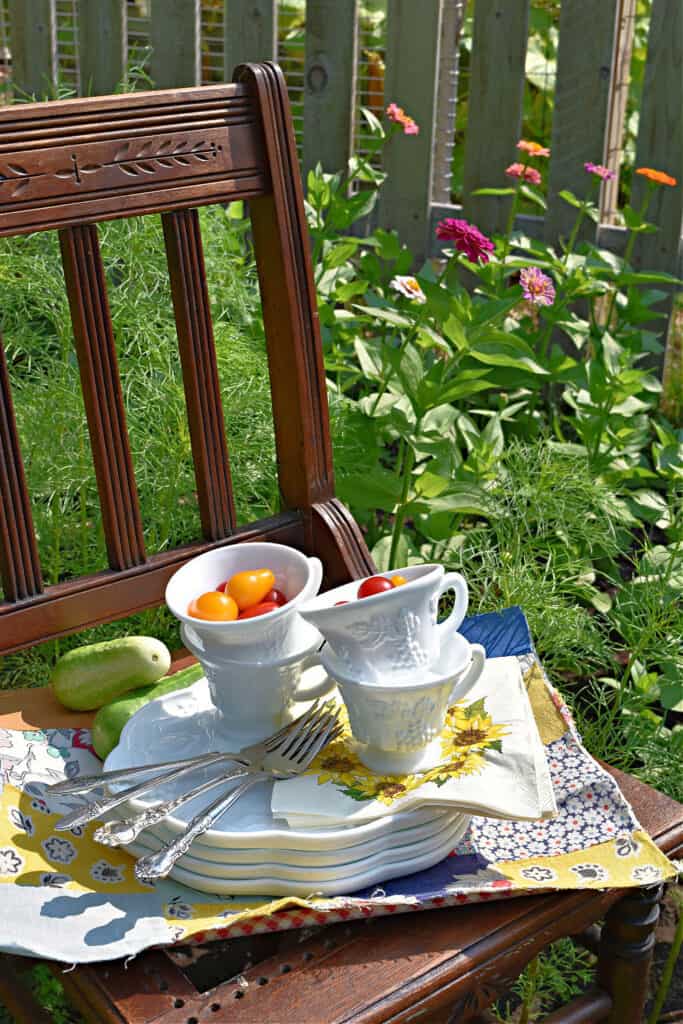In this portrait-oriented outdoor image, we see an ornate, wooden chair positioned slightly cut off on the left foreground. The chair boasts intricate carvings, including a detailed leaf motif across the top back, hinting at its antique charm. Draped over the chair is a folded, multicolored tablecloth featuring a vibrant mix of yellow, grey, and white flowers with orange centers. Resting atop the tablecloth is a set of plates, creatively shaped like clouds or flowers, presenting a whimsical touch. On these plates, we see four white china teacups, stacked in pairs, each filled with heirloom tomatoes in hues of red and orange.

Adjacent to the teacups, a couple of elongated green courgettes lay nestled, adding a fresh touch to the arrangement. Beneath the teacups on the right, white napkins adorned with cheerful yellow daisies peak out. Forks with ornate silver designs are placed with their handles pointing leftward, completing the elegant setup. Surrounding this pastoral scene are lush, rough foliage and tall carnations standing in shades of dark and light pinks as well as oranges. Behind this vibrant flora, a light pine wooden fence, intertwined with chicken wire, can be seen, with indistinct brownish objects lurking behind it. This carefully curated display suggests the anticipation of a delightful garden tea party amidst the verdant beauty of nature.